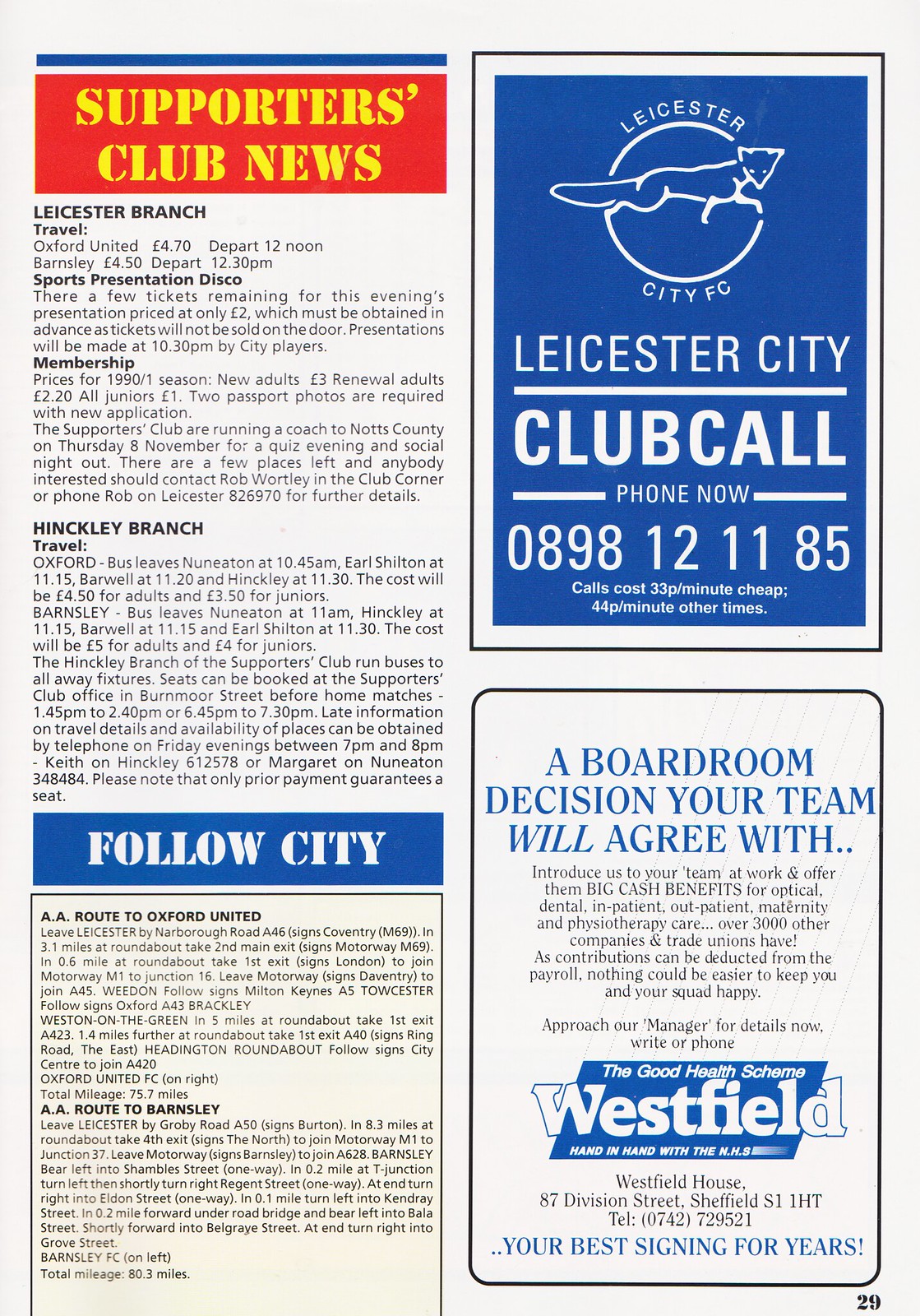This detailed page appears to be from a sports magazine or game day program, printed on white paper with a page number "29" in small print at the bottom right corner. The layout is divided into two columns. In the top left corner, a red rectangle with bold yellow text announces "Supporters Club News," followed by sections about the Leicester and Hinkley branches, including travel information. Midway down the left column, a blue box with white letters reads "Follow City," detailing AA routes to Oxford United and Barnsley. The right column features two advertisements. The top ad promotes the "Leicester City Club Call" with a phone number "0898-121-185" and additional fine print. Below, a second ad, featuring a blue rectangle, states, "A Boardroom Decision Your Team Will Agree With," highlighting Westfield’s collaboration with the NHS and describing it as "your best signing for years."